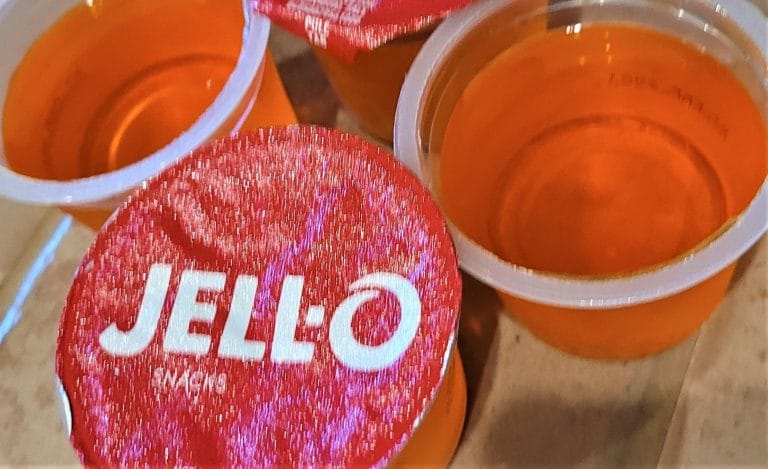The photograph captures four containers of Jell-O arranged in a diamond formation on a light brown surface, possibly a table or piece of cardboard. Two of the containers—positioned at the top and bottom of this diamond—still have their red foil lids intact, displaying the iconic Jell-O logo with "snacks" written below. The other two containers, on the left and right, have their lids peeled off, revealing untouched orange-colored Jell-O inside. The image is slightly blurry, suggesting it was taken with a smartphone or a lower-quality camera, and is cropped to a widescreen aspect ratio, cutting off a portion of the top container. The orange hue of the Jell-O indicates they are likely orange-flavored, although no specific flavor text is present.